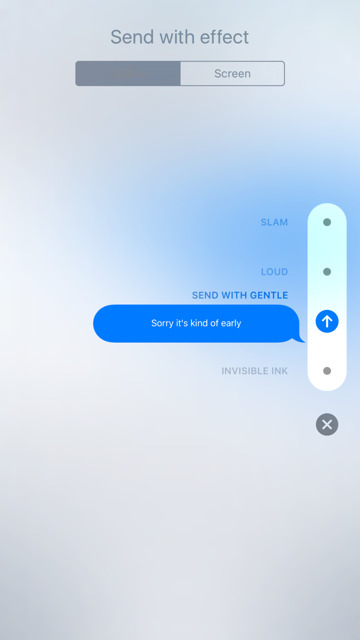The image features a gradient background that transitions from light purple on the edges to light blue toward the center. At the top, the word "Slam" is prominently displayed in gray. Below this, there is text that reads "Sin with Effect." Underneath the text, a rectangular box is split into two halves; the left half is filled in gray while the right half remains uncolored. Centered within this box is the word "Green."

On the right side of the image, there is an oblong white button featuring two small gray circles at the top and one at the bottom. Above the bottom circle is a larger blue circle with an arrow pointing up and down. Below this, a gray circle contains an 'X' in the middle.

To the left of this white oblong button, the word "Slam" appears again at the top, followed by a space, then the word "Loud" in the middle. The phrase "Sin with Gentle" is displayed beneath this, and next to it, a blue text box contains the message "Sorry it's kind of early." Finally, at the bottom, "Invisible Ink" is written.